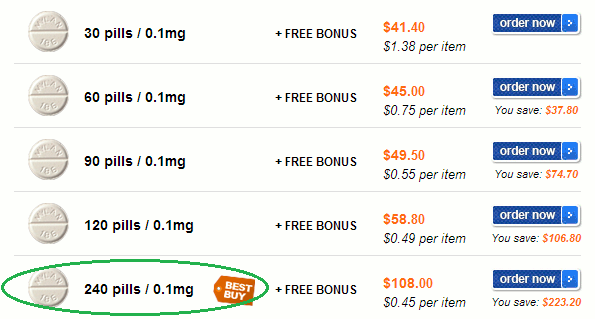The website offers various purchasing options for 0.1 mg pills, displaying the price and savings for bulk orders alongside clear images and order buttons. 

1. The first option showcases 30 pills at 0.1 mg each, pictured as basic white tablets with a bisecting line. A free bonus is offered, with a total price of $41.40 in orange text ($1.38 per pill in black). A blue "Order Now" button is available next to this option.

2. The second option features 60 pills with the same image and dosage. The displayed price is $45.75 ($0.76 per pill) with a free bonus. You can order this quantity using the blue "Order Now" button.

3. The third option is for 90 pills at the identical dosage and image. It includes a free bonus and is priced at $49.50 ($0.55 per pill). The blue "Order Now" button is also present here.

4. The fourth option lists 120 pills of the same dosage and image, offering a free bonus. The total cost is $58.80 ($0.49 per pill), with an adjacent blue "Order Now" button.

5. The final option, highlighted with a green circle and an orange "Best Buy" tag in white letters, is for 240 pills. The price is set at $108.00 ($0.45 per pill) and includes a free bonus. This option also features a blue "Order Now" button.

Each option indicates potential savings when purchased in bulk.